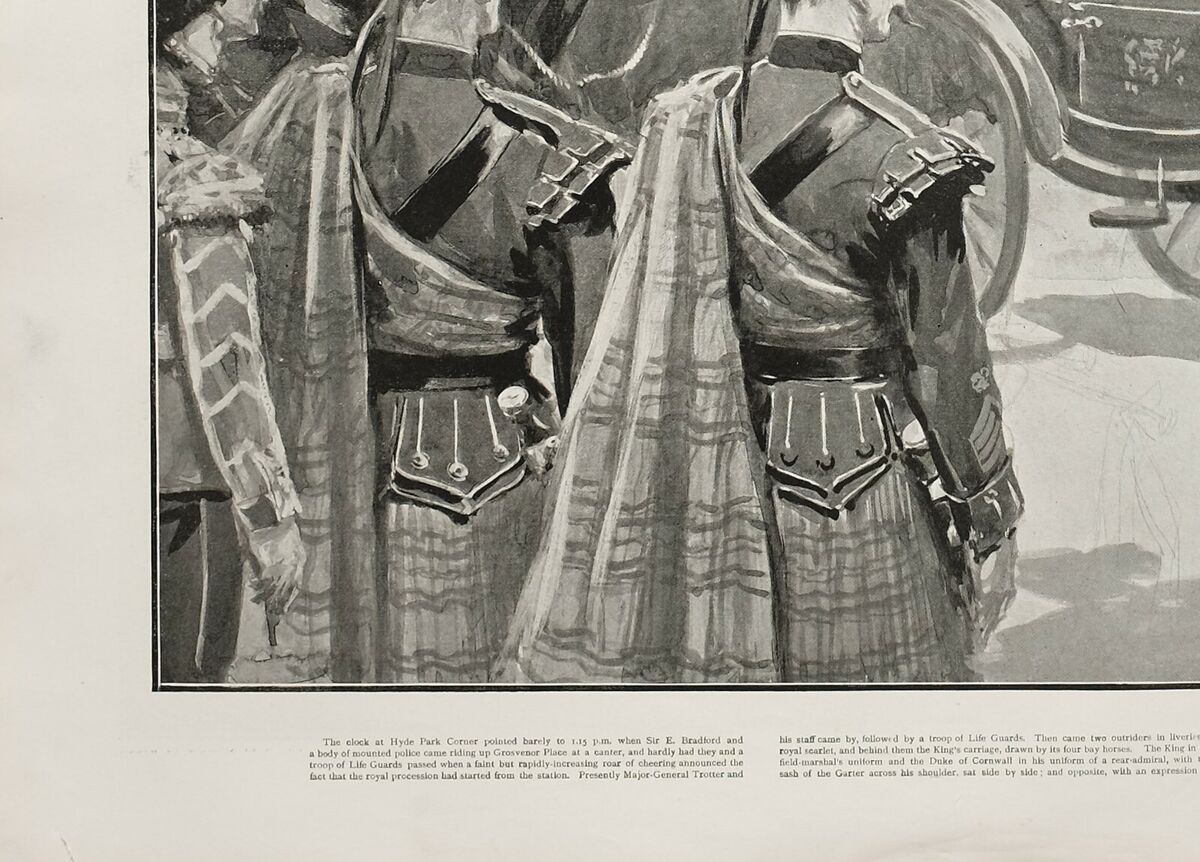The image appears to be a black-and-white illustration, possibly a watercolored drawing, taken from a page on light gray stock, perhaps from a book. The dominant feature is the rear view of two soldiers, likely from the Highland Regiments, both adorned in plaid kilts with matching cloaks draped over their left shoulders. They are equipped with Sam Browne belts and black bandoliers, and bear epaulets and black collars. The rightmost soldier, distinguished by an elaborate mustache and sergeant stripes on his arm, stands adjacent to a horse carriage, of which only the bottom and a few wheels are visible. Below the illustration, a block of small text provides further description, although it is partly cut off and unreadable. The entire image is incomplete, with sections truncated on the right and at the top.